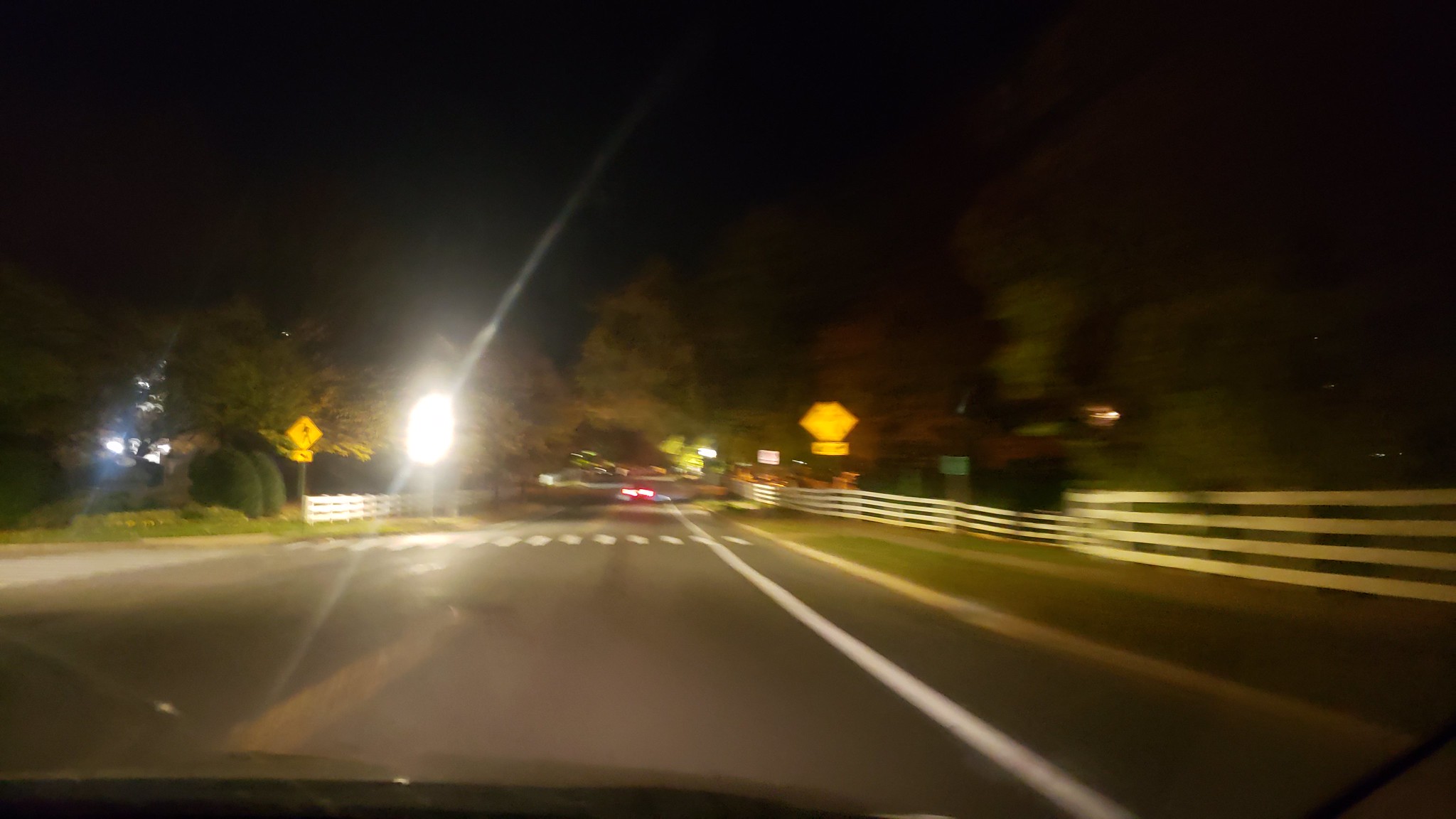This nighttime image, captured from the passenger seat of a car via a dash cam, depicts an American two-lane road. The foreground features part of the vehicle's windshield and hints of the car's interior, reflecting light from an external source. The road, paved with gray asphalt, is lined with various markings: a solid white line on the right, double solid yellow lines on the left, and a pedestrian crosswalk distinguished by its solid vertical white lines. In the distance, the blurry red taillights of another vehicle are visible. The scene is framed by white picket fences on both sides, with a sidewalk on the right. A diamond-shaped yellow pedestrian crossing sign is prominently displayed on the left-hand side, illuminated by a nearby light. Surrounding the road, tall trees, green grass, and bushes add a natural contrast to the man-made elements. There is a branching road to the left after the crosswalk, adding depth to this nocturnal street view.